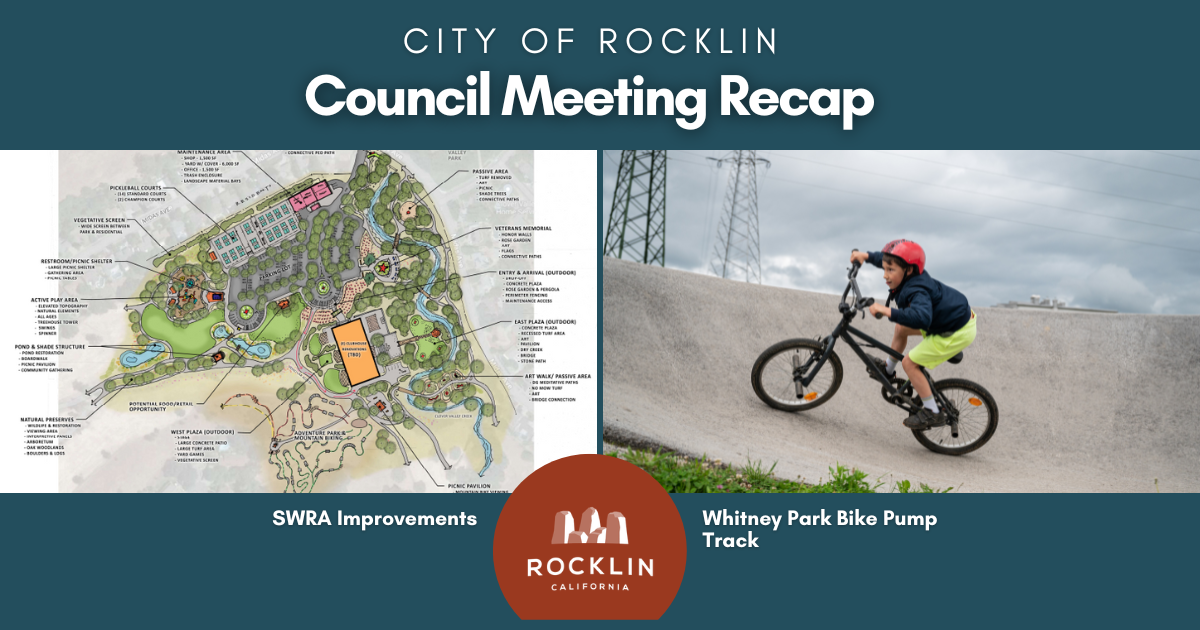This rectangular landscape image from an online site is advertising a council meeting recap for the City of Rocklin. The background is divided into two thick, darker bluish-green sections, top and bottom. At the top, in white capital letters, it reads "CITY OF ROCKLIN," and below that, in a larger bold font with initial capitals, "Council Meeting Recap." 

Centrally, at the bottom, there is a partially visible red circular logo. Within this logo, in white capital letters, it says "ROCKLIN," with "CALIFORNIA" below it, featuring a drawing of mountains above the word "ROCKLIN."

On the left side of the image, there's a detailed, irregularly shaped, drawn map of Rocklin. This map is filled with green trees, various buildings, small text, and arrows pointing to different parts. A prominent feature within this map is an orange rectangular area. Beneath this map, in white capital letters against the blue-green background, it reads "SWRA IMPROVEMENTS."

To the right, a photograph shows a young boy, aged around 8 to 10, riding a black bike with handlebars in a bike park. He wears a red helmet, a long-sleeve blue shirt or sweatshirt, neon light yellow-green pants, black sneakers, and white socks. The boy is biking on a curved grey track. Behind him are two large power lines and a patch of grass. Below this photo, it says "WHITNEY PARK BIKE PUMP TRACK" in white letters against the blue-green background.